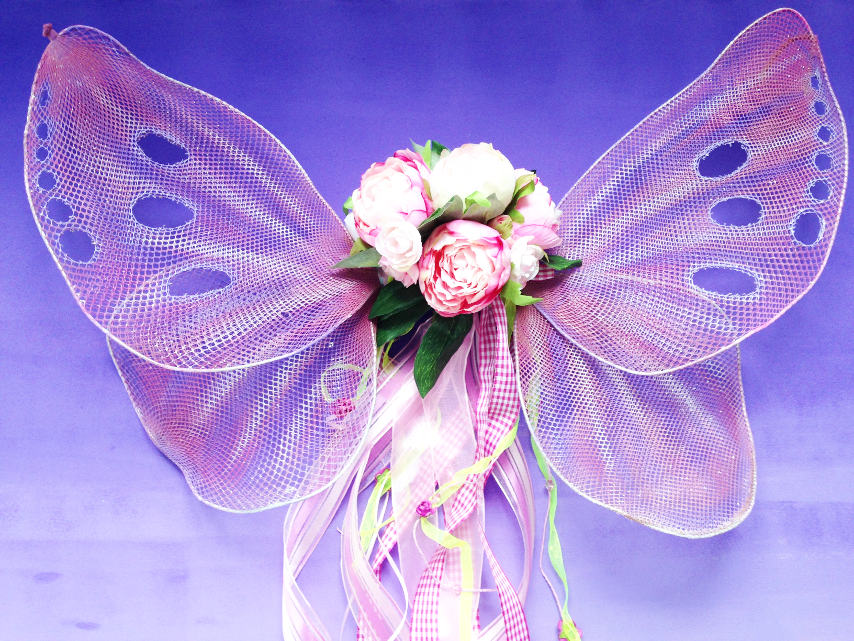This image showcases a whimsical corsage of flowers artistically arranged to resemble a butterfly, set against a purple background. The flowers are tied together with a variety of colorful ribbons, including pink and white plaid, yellow with pink accents, light green, and white ribbons of different thicknesses. Notably, there is a distinctive striped ribbon featuring two thick white stripes flanking a thick pink stripe in the center. The "wings" of the butterfly are crafted from a netting material with intricate holes, giving them a slightly transparent appearance. This creative arrangement combines elements of natural beauty and fantasy, almost making it look like a digitally drawn graphic rather than a real object. With its vivid ribbons trailing down and detailed netting wings, this flower corsage beautifully mimics the whimsical and delicate form of a butterfly.